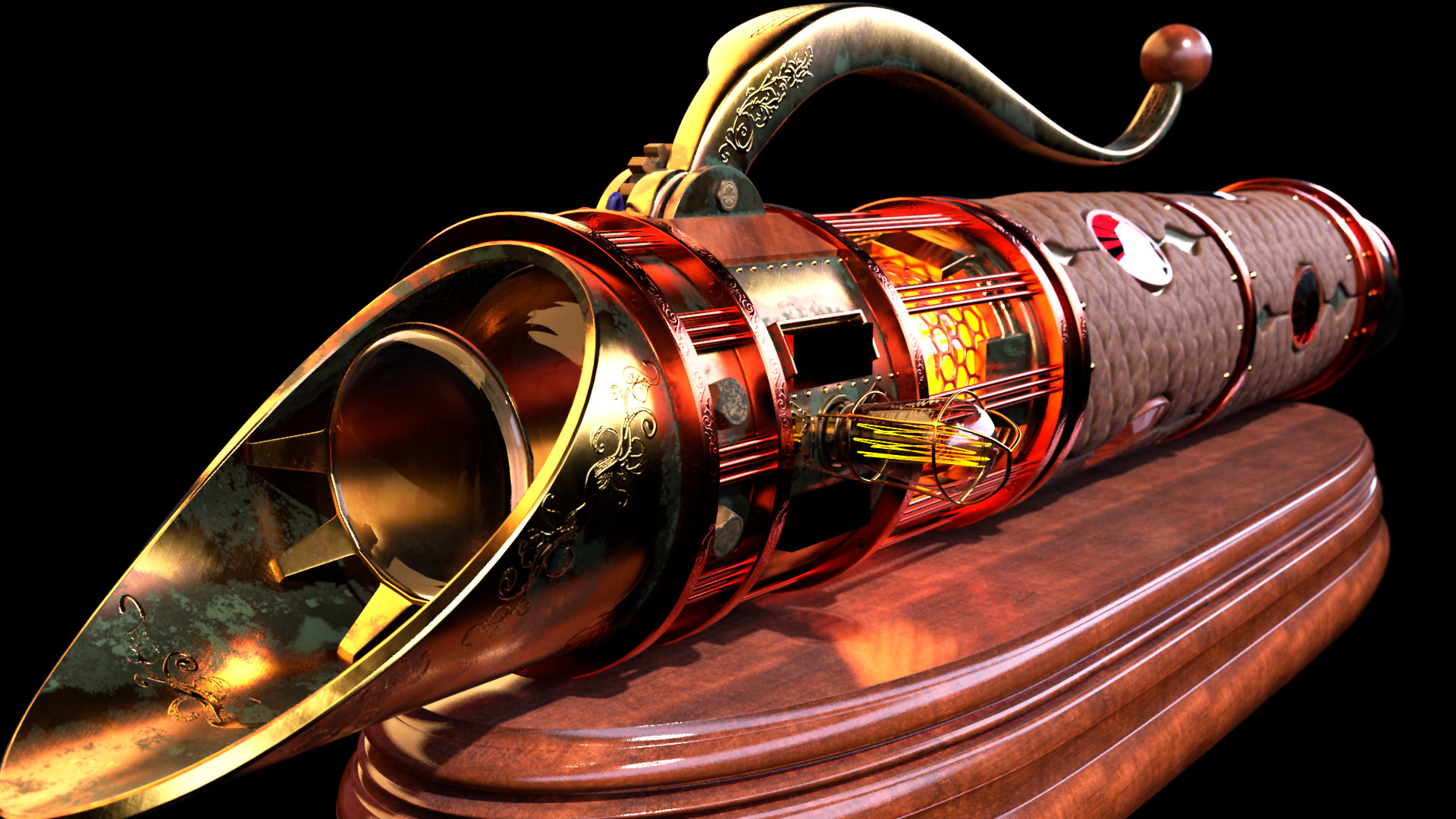This image depicts a computer-generated rendering of a long, cylindrical object, evocative of both a musical instrument and an antiquated lightsaber hilt from Thomas Edison’s era. The setting presents a stark contrast, with the object resting on a wooden plaque against an entirely black background. The object is vividly colored in hues of red, yellow, orange, and white, featuring intricate designs. The front end, gold in color, has an oblong opening leading to another cylinder with its own opening. Near the front, an old-timey filament light bulb protrudes to the side. The object also boasts a slick, waved handle at the top, which extends into a tail-like figure accented in yellow and beige, culminating in a burgundy brown ball. Towards the back, a quilted purple pattern is adorned with circular gauges and windows, adding to its intricate and antique appearance.